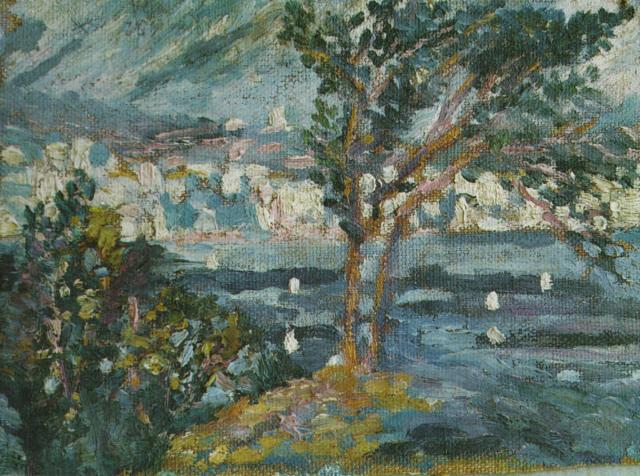The painting showcases a thin brown tree with an array of dark green leaves prominently positioned at the center, surrounded by a body of water. To the bottom left, a green bush with various leaves adds to the lush scenery. The water, primarily light blue, is dotted with white, possibly indicating plant life. Above the water is a striking white cliff side, adorned with various splotches of blue, extending from right to left across the image. The sky, painted in a light blue hue, is speckled with patches of dark blue, adding depth and contrast. The entire scene is rendered in a blotchy, impressionistic style, characterized by strokes and swatches of color, capturing the natural elements in an abstract, non-realistic manner.